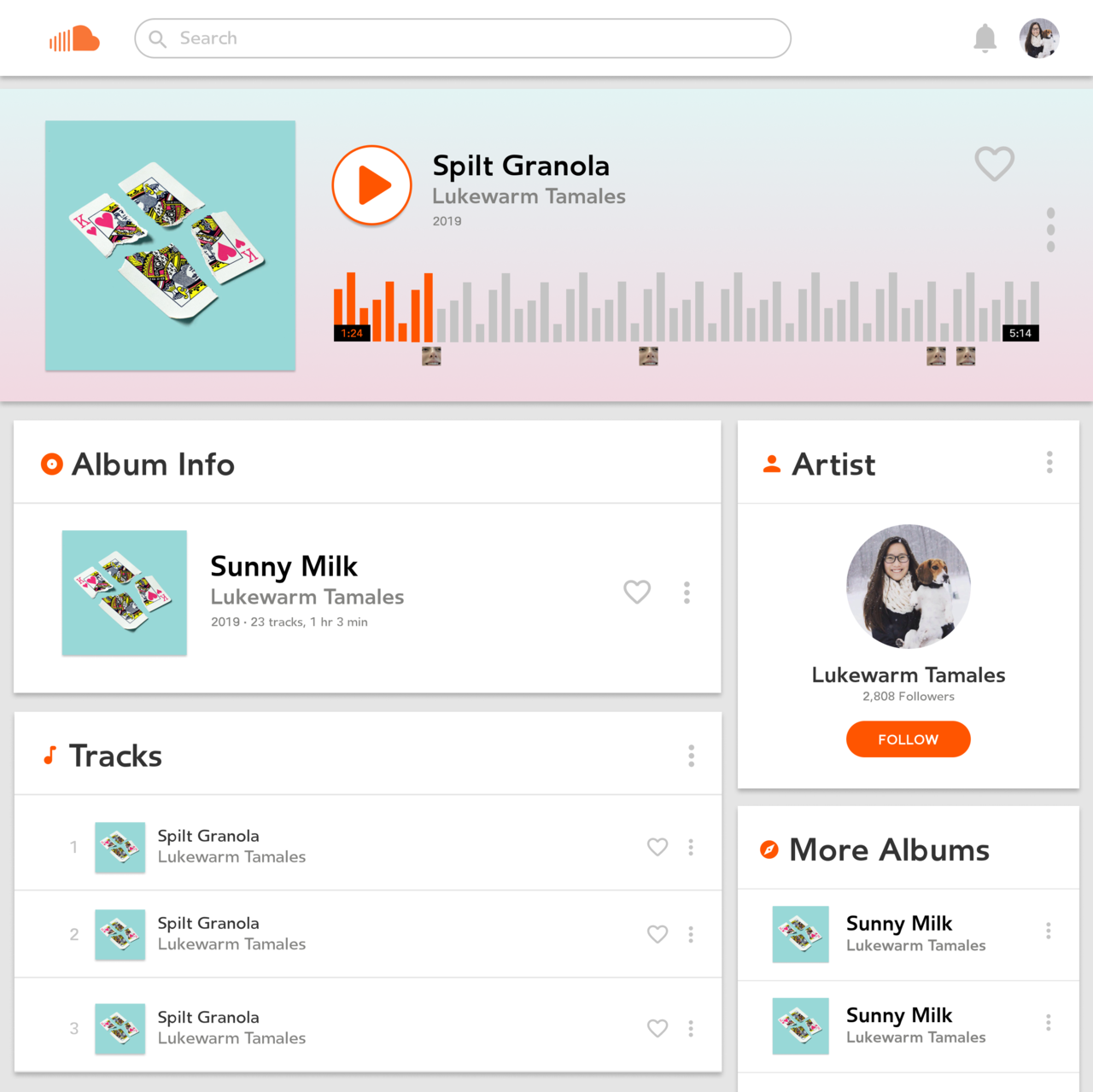The image depicts a square web page featuring a music website interface. At the top, there's an orange cloud with lines radiating behind it, symbolizing the site's logo. To the right, there is a search bar and a user profile icon depicting a woman. Just beside the profile icon, there's a notification bell.

Below this top section, a horizontal banner with a gradient background transitioning from pink to blue captures attention. On the left side of this banner, there's a square image of a blue background featuring a King of Hearts card torn into four pieces. Next to the image is an orange arrow encircled in orange, indicating the currently playing song.

The song displayed is "Split Granola" by Lukewarm Tamales. Beneath the song title, there's a progress bar consisting of vertical bars; the first nine bars are highlighted in orange, indicating the song's progression, while the remaining bars are gray. Smaller square icons displaying faces are positioned below this bar.

On the left side, beneath this progress bar, is the album information section. It mirrors the torn King of Hearts card image from above and lists the album title as "Sunny Milk" by Lukewarm Tamales. The tracklist shows "Split Granola" repeated for tracks 1, 2, and 3.

To the right of the album information, there's a box labeled "Artist" containing a more detailed version of the profile picture. It shows a woman smiling while holding a dog out in the snow, indicating a personal connection to the artist, Lukewarm Tamales, who has 2,808 followers. A follow button is available just below this section.

In the lower right corner of the page, a "More Albums" section features additional albums titled "Sunny Milk" by Lukewarm Tamales.